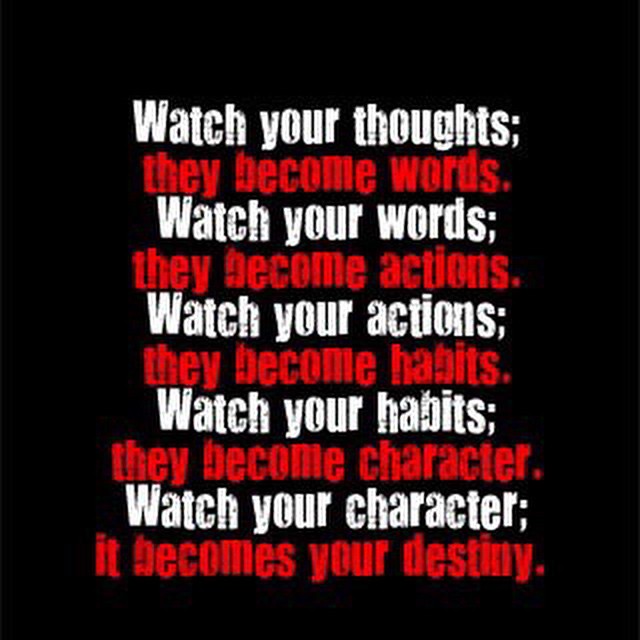The image is a slightly taller than wide poster with a completely black, degraded background, giving it a worn-out appearance. Centered in the middle are several lines of text that alternate in color between white and red. The white lines begin with motivational phrases starting with "Watch your," followed by red lines that complete the thoughts. The text reads: 

"Watch your thoughts; they become words. Watch your words; they become actions. Watch your actions; they become habits. Watch your habits; they become character. Watch your character; it becomes destiny."

Each phrase starts in white and concludes in red, with a semicolon separating the parts of the phrases, except the final line which ends with a period. The text is slightly worn, adding to the poster's vintage feel. There is no attribution or further context provided.